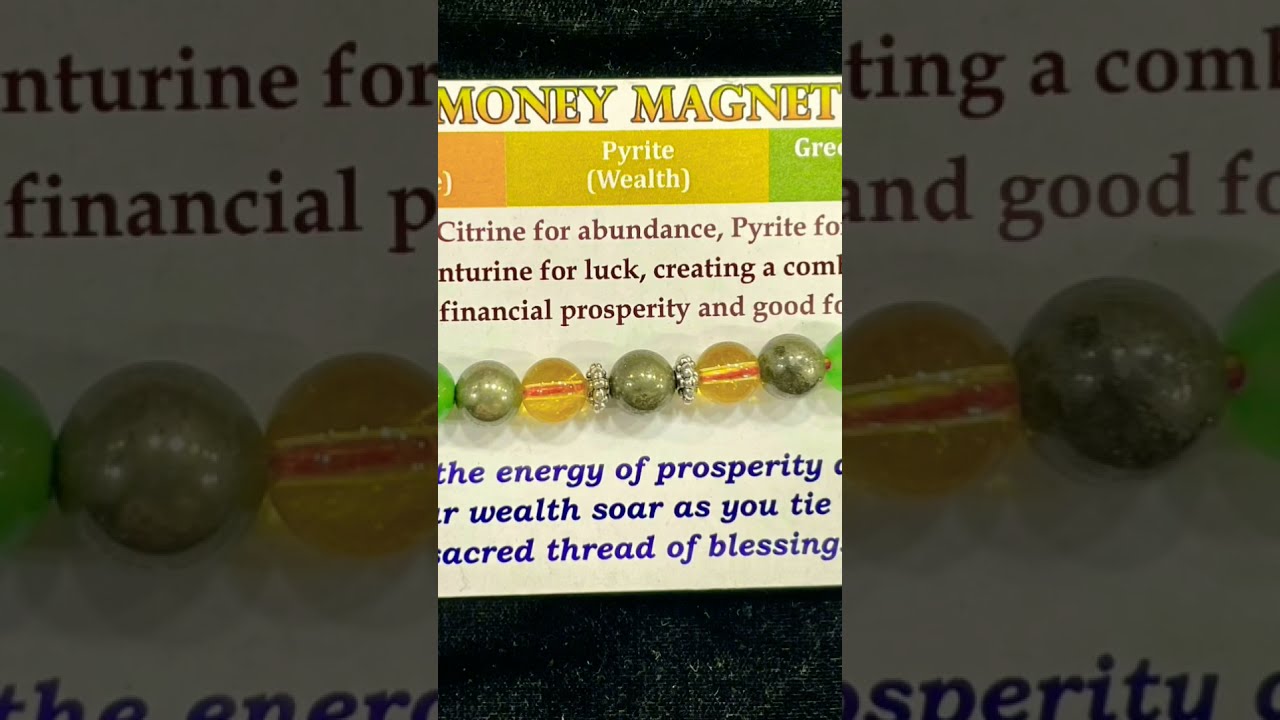The image features a horizontally aligned rectangular box segmented into three panels. The central panel is bright and clear, showcasing an array of beads or possibly a bracelet with stones of varying hues—green, gold, and pewter. At the top of this middle section, "Money Magnet" is prominently displayed in yellow letters. Beneath it, a series of colored bands (peach, yellow, and green) are visible, each marked with text. The text within the bands includes "Pyrite (wealth)" in yellow, followed by partially obscured phrases indicating that citrine is for abundance, and pyrite confers financial prosperity. Text at the bottom section of this panel, although partially cut off, mentions "financial prosperity and good fortune," concluding with the phrases "the energy of prosperity," and "sacred thread of blessing" in blue letters. The left and right panels, darker and shadowed, mirror each other, containing partial close-ups of the same images and text seen in the middle panel. The repeated items and text appear slightly more legible in these sections, though the cut-off text still obscures some details.